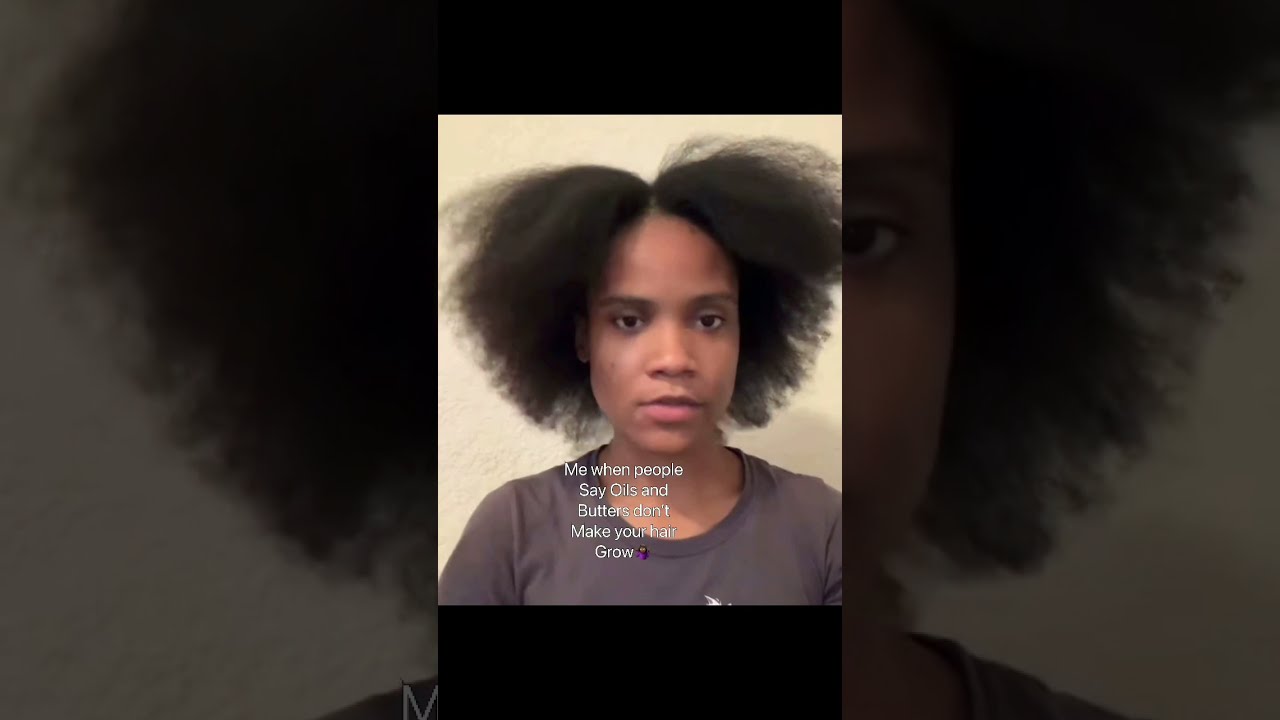The image features a photograph of an African American woman with brown skin, who is facing the camera with a neutral, unamused expression. Her naturally poofy hair, either very dark brown or black, parts down the middle and extends to her chin, framing her face. She has wide, dark eyes, a broad nose, and distinctively large, pinkish lips. The woman wears a shirt that appears to have a gray-purple tone and possibly a graphic that fades toward the bottom of the frame. There's a text overlay in white font on the image that reads, "Me when people say oils and butters don't make your hair grow," accompanied by a small, purple emoji. This image also serves as the backdrop, but in a darkened and blurry form, emphasizing the clarity and vibrant colors of the main picture. The woman is seated in front of a plain white wall, and this focused, detailed portrait captures her direct eye contact with the camera.